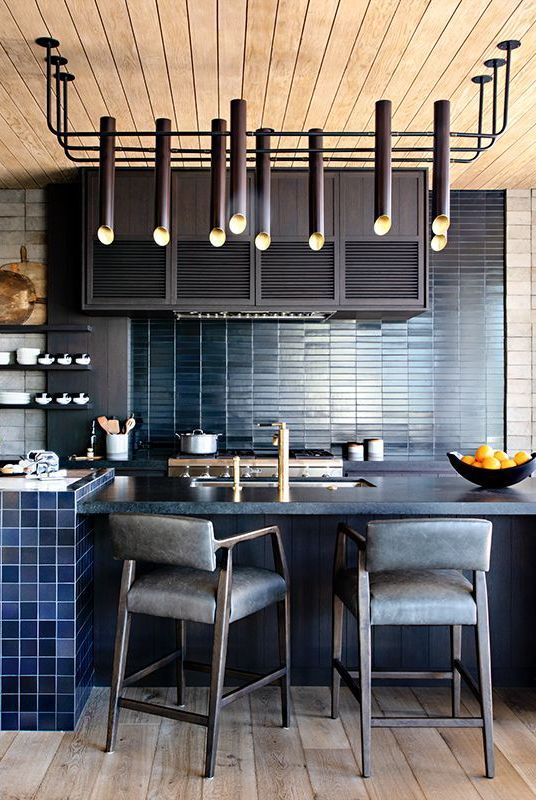This highly professional and modern kitchen interior resembles something out of a home and garden or interior design magazine. The sophisticated space features light brown wooden plank flooring that adds warmth to the room. An island area, centrally located, boasts a luxurious dark marble countertop with a recessed sink. A sleek black bowl filled with oranges sits to the right, alongside two tall black leather stools. 

To the left of the island, a counter made of 6x6 inches mosaic blue tiles adds a splash of color and dimension. The kitchen's back wall is adorned with a refined thin navy tile, providing continuity to the blue theme. Adorning the wall are dark-colored cabinets, complemented by black floating shelves displaying an array of neatly organized white plates and dishes. 

Above the stainless steel stove, there's a black wooden cupboard, further enhancing the kitchen's dark theme. The ceiling, composed of brown wooden planks, is accented by tube-like lights that hang creatively, almost resembling bamboo shoots. This detailed and cohesive design presents a stylish and inviting kitchen space, perfect for any high-end home or professional listing.